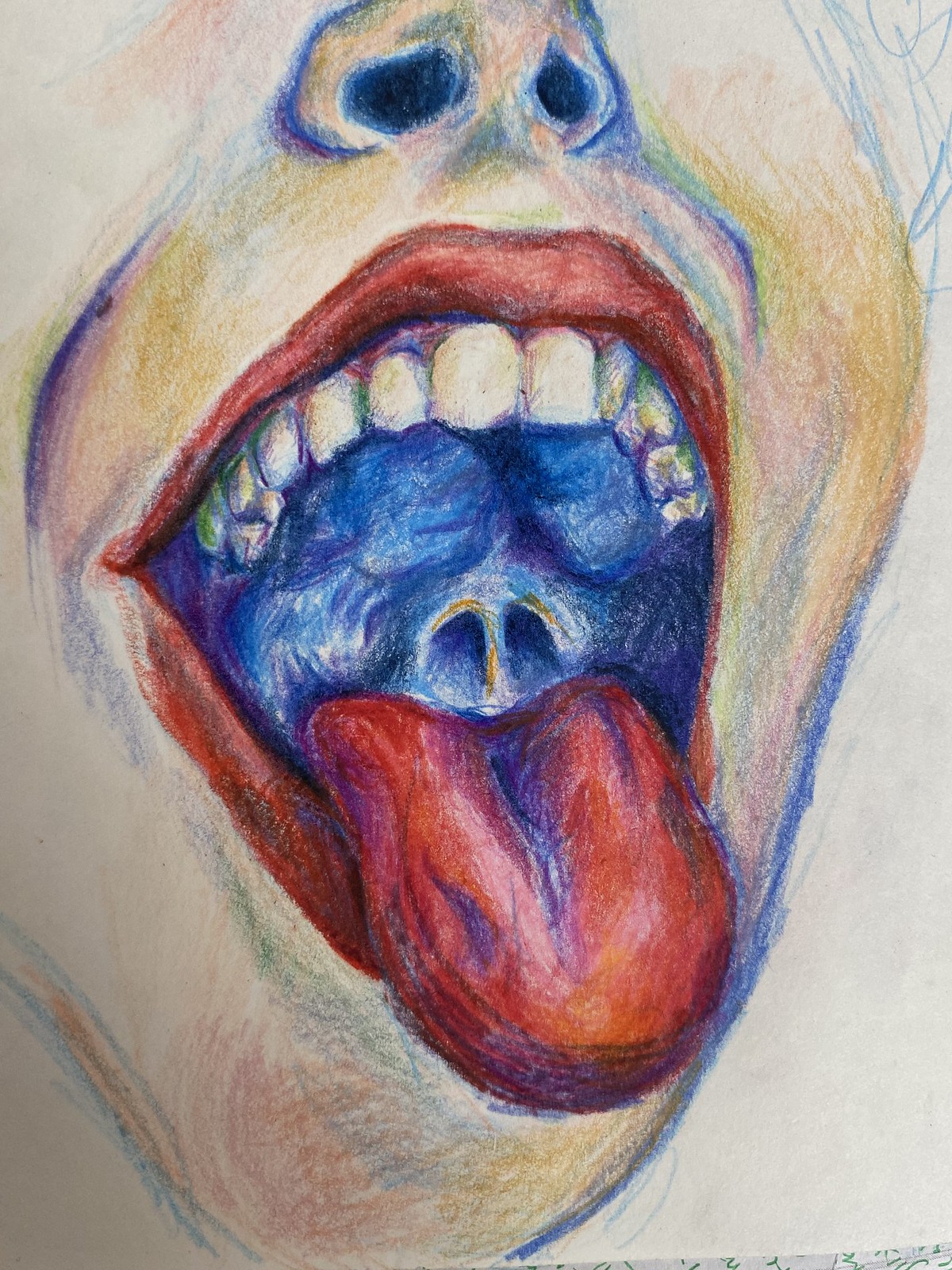This detailed illustration on white art paper captures the bottom half of a human face, focusing predominantly on a wide open mouth. Rendered with colored pencils and pastels, the drawing is strikingly realistic. The mouth, accentuated by vividly red lips—suggestive of lipstick—and a bright red tongue, commands attention. The tongue protrudes outwards, obscuring the bottom row of teeth while revealing a clear view of the upper teeth and trailing down to cover a part of the chin. The mouth's interior is shaded in blue, simulating darkness and depth, with visible anatomical details such as the throat, tonsils, and the epiglottis. The depiction extends upwards to the nostrils of a clipped nose, showing dimple lines on one side. This art piece, through its rich use of color and meticulous detailing, vividly encapsulates the intricacies of the human mouth in a moment of wide-open expression.